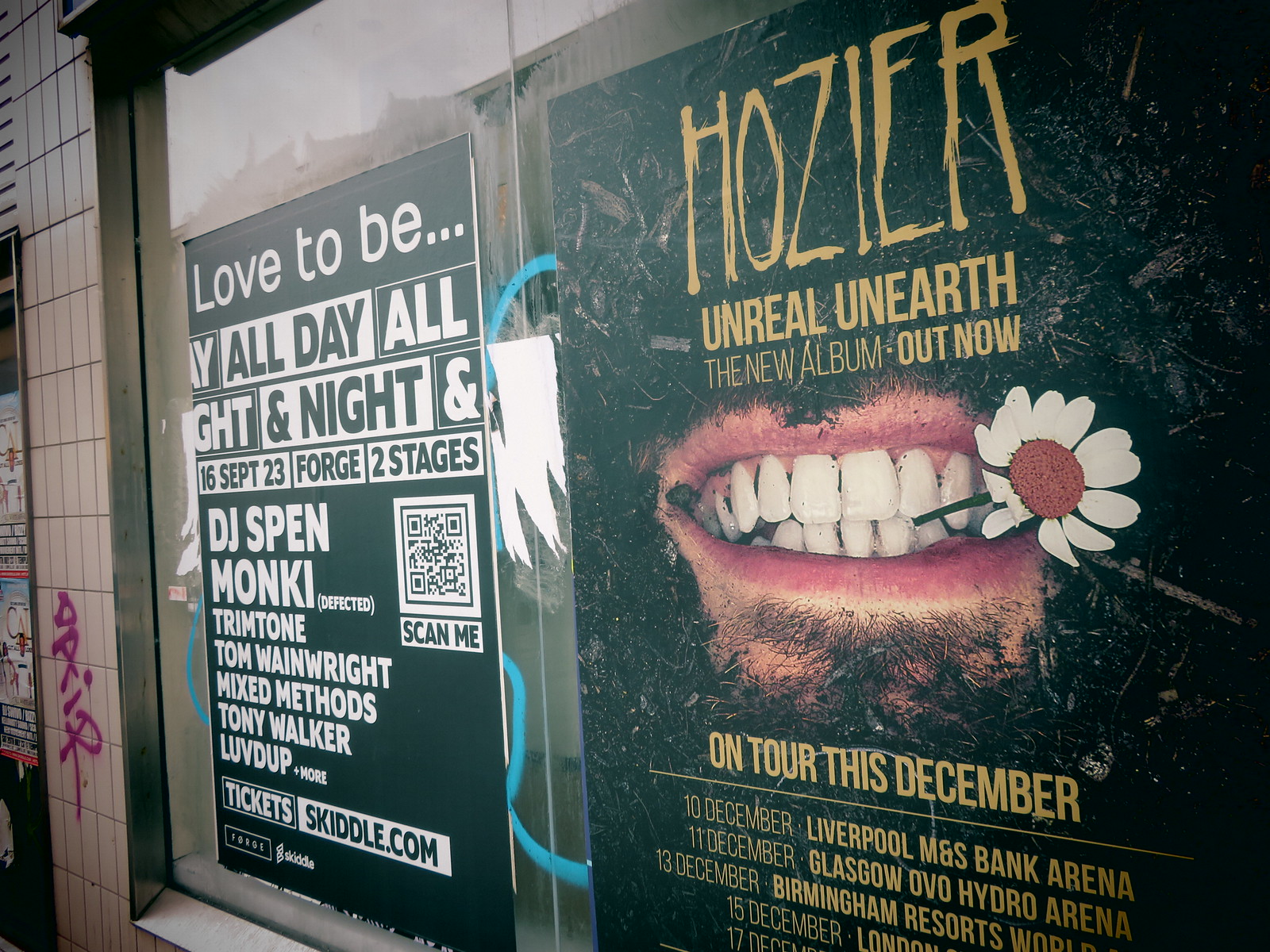This image, taken outdoors during the daytime, depicts the windows of a shop storefront arranged in a rectangular frame that is wider than it is tall. Primarily on the right-hand side, we see a large black poster featuring gold text that reads "Hozier." Below this, it announces "Unreal Unearthed, the new album out now." The poster includes a close-up photograph of a man's mouth, clenched teeth holding a fancifully drawn daisy, with some facial hair visible beneath the lower lip. Additional gold text below the image details an upcoming tour: "On Tour This December," listing dates and venues including 10th December at the Liverpool M&S Bank Arena, 11th December at Glasgow OVO Hydro Arena, 13th December at Birmingham Resorts, and 15th December in London. 

To the left of the Hozier poster is another black background poster with white text, promoting an event called "Love to Be." It includes phrases such as "All Day, All Night," and indicates dates and lineup details: "16th September 23rd, Forge II Stages, DJ Spendmonkey, Trim Tone, Tom Wainwright, Mixed Methods, Tony Walker, Loved Up.” There is also a mention of ticket availability at "Ticketskittle.com" and a barcode labeled "Scan Me."

Further left, the storefront’s backdrop becomes visible: a brown-tiled wall, marred by pink graffiti displaying the tag "D-A-I-R." This section of the wall suggests a spot that has repeatedly hosted various posters and advertisements over time, adding a grungy, layered aesthetic to the scene.